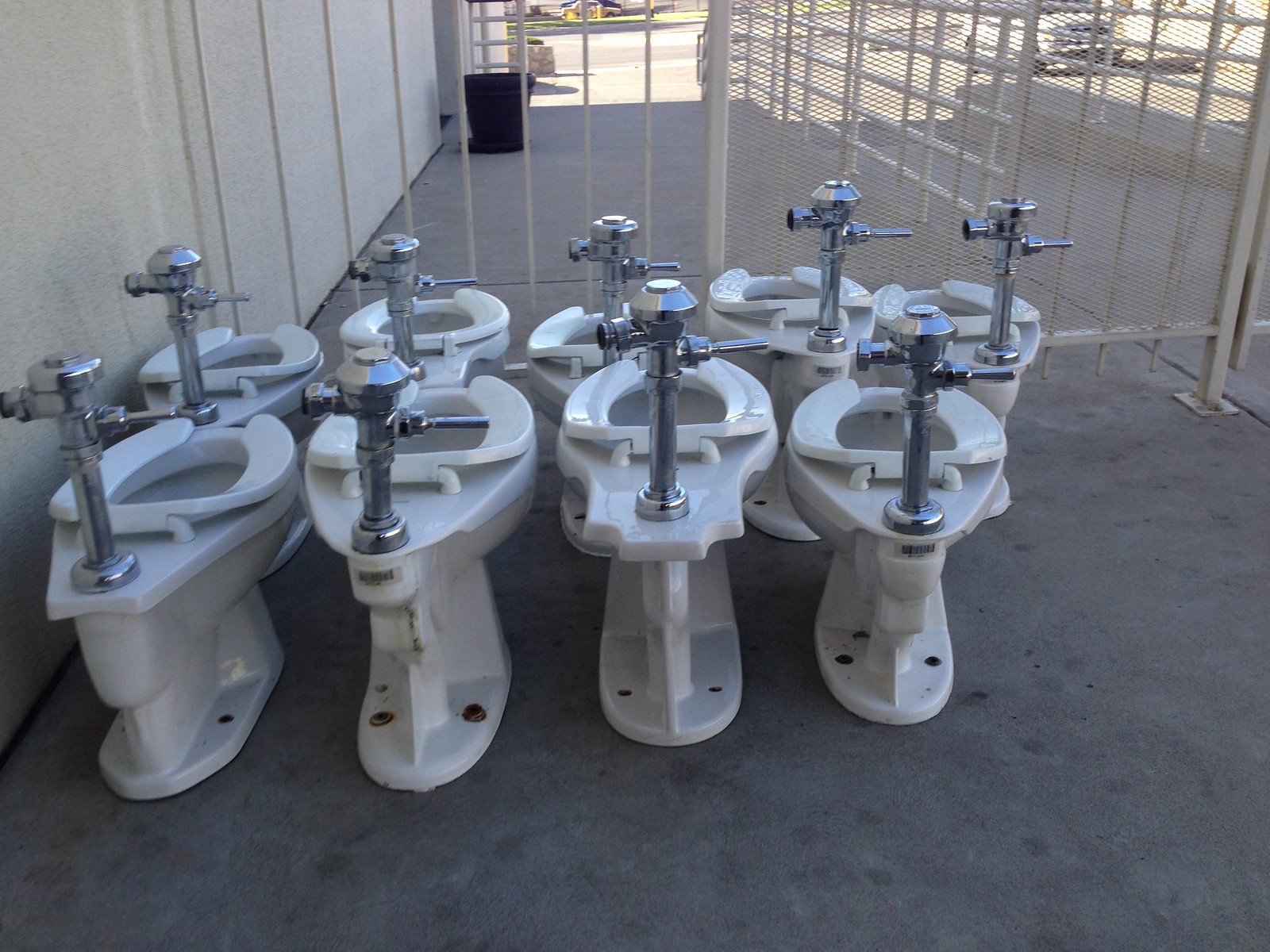This color photograph captures an outdoor area adjacent to a building, featuring a collection of nine white porcelain toilets, arranged in two neat rows—four in the front and five behind. The perspective shows the back of the toilets, each equipped with a chrome flush handle and lacking an upper tank. These toilets appear to have been removed from a commercial or public restroom, evident from their utilitarian design and slight wear. They stand on a concrete or asphalt surface and are enclosed by a metal cage, resembling a prison-like storage space designed to protect them. In the background, through the wire fencing, a sunny street with a parked white car is visible, emphasizing the juxtaposition of the shaded storage area and the bright external environment. The entire scene suggests a makeshift storage or refurbishment yard temporarily housing these fixtures.